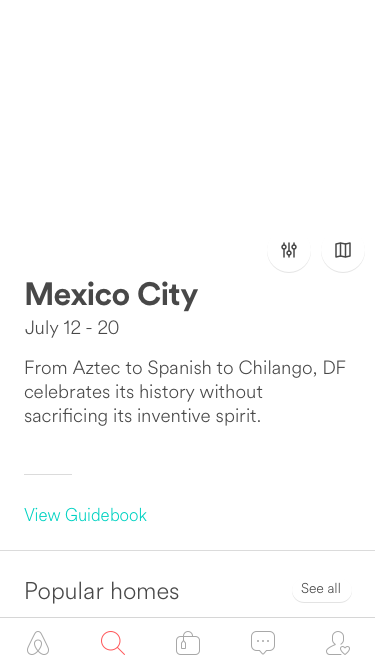The image features the following elements:

- In black text, "Mexico City" is prominently displayed.
- To the right of "Mexico City," there are three vertical lines:
  - The first and third lines each have a circle at the top.
  - The middle line has a circle in the middle.
- Further to the right, there is a square with horizontal and vertical lines inside it.
- Below "Mexico City," the dates "July 12th through 20th" are listed.
- Under the dates, the text reads: "From Aztec to Spanish to CHILANGO, D.F. celebrates its history without sacrificing its inventive spirit."
- Approximately four inches below this text, there is blue text stating "View guidebook," followed by a long horizontal light gray line.
- Below the line, the section titled "Popular Homes" appears with a "See All" option to the right.
- Under "Popular Homes," the Airbnb logo is displayed, which is a triangular design meeting in the middle, alongside a red magnifying glass representing a search function, a suitcase icon indicating shopping with a tag hanging on its side, a speech bubble containing three small dots, and an image of a person's silhouette accompanied by a small heart.

This detailed caption helps in visualizing the layout and the contents of the image accurately.